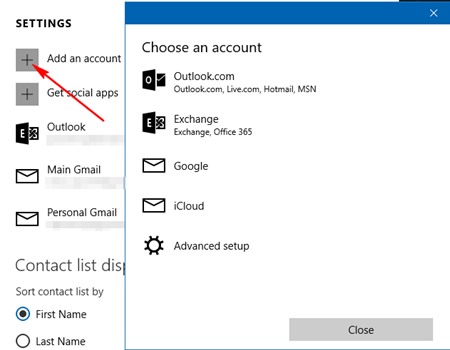Screenshot of a digital device screen displaying a settings menu. The exact device type is indeterminate but could be a computer, smartphone, tablet, or Kindle, evident from the digital nature of the interface. The menu features several options prominently:

1. A section titled "Settings" at the top with a plus sign next to "Add an Account", highlighted by a red arrow pointing diagonally upwards.
2. Directly below, another option with a plus sign labeled "Get Social Apps".
3. An icon for Outlook is present followed by an envelope icon labeled "Main Gmail" and another envelope icon beside "Personal Gmail".
4. Additional settings include "Contact List Display" with a submenu titled "Sort Contact List By", where "First Name" is selected over "Last Name".
5. A white rectangular area with a blue header titled "Choose an Account" listing five icons down the side for Outlook.com, Exchange, Google, iCloud, and Advanced Setup.

The overall interface suggests this could be an account management or contact settings screen on a digital device.